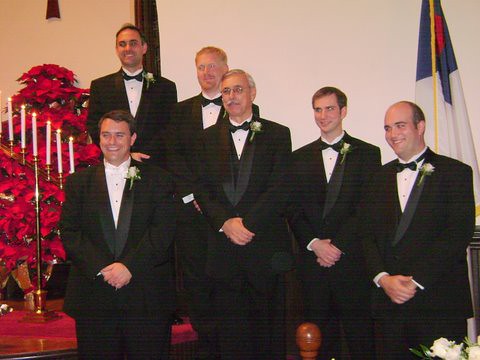This image appears to capture a moment from a wedding or ceremony. It features six men wearing tuxedos with black bow ties, except for the one standing in front who sports a distinct white bow tie. Each man has a white rose pinned to his lapel. They are all posing, smiling, and looking towards the camera, their hands held in front of them. The indoor setting has a fairly white background with a notable black pillar on the left. Red poinsettia plants and a tall gold candlestick holding six lit white candles are also visible. Additionally, a flag with a blue upper corner and a predominantly white body can be seen in the upper right corner.